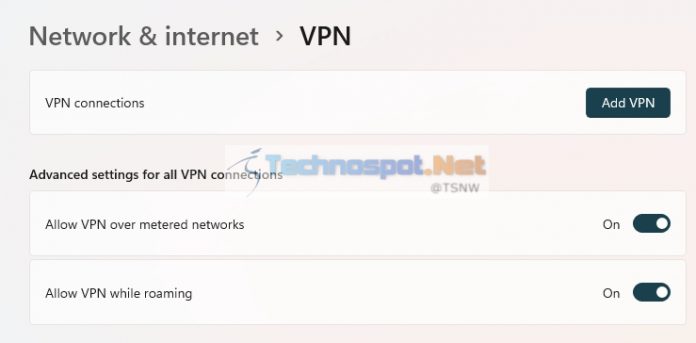The image showcases a rectangular landscape-shaped screen approximately twice as wide as it is high, set against a light cream background with a subtle hint of pink. In the upper left corner, "Network & Internet" is displayed in gray text, with only the "N" in "Network" capitalized. Following this text is a right-facing arrow tip symbol, leading to "VPN" in bold black font.

Beneath this heading are three long, white rectangles extending nearly the full width of the image. The first rectangle, directly below the header, has "VPN connections" written in gray text on the left. On the far right of this rectangle is a smaller, dark blue button with rounded corners, labeled "Add VPN" in white text, indicating a clickable option to add a VPN connection.

Below this section, there is a small gap before the next header, "Advanced settings for all VPN connections," displayed in smaller, bold black font. Underneath, two additional white rectangles provide further settings options. The top rectangle reads "Allow VPN over metered networks" on the left, and the one below it states "Allow VPN while roaming," both in dark gray text. To the right of each of these settings are blue toggles, shaped like rectangles with curved sides, each with a white circle on the right side indicating the current "on" position. The toggles can be switched off by moving the white circles to the left.

Centrally placed in the image is a watermark reading "technesspot.net," with "dot net" colored in a yellowish-orange. The watermark text is modest in size, comparable to the "Network & Internet" text in the upper left corner. Overall, the watermark is small and unobtrusive, ensuring it does not detract from the primary content of the image.